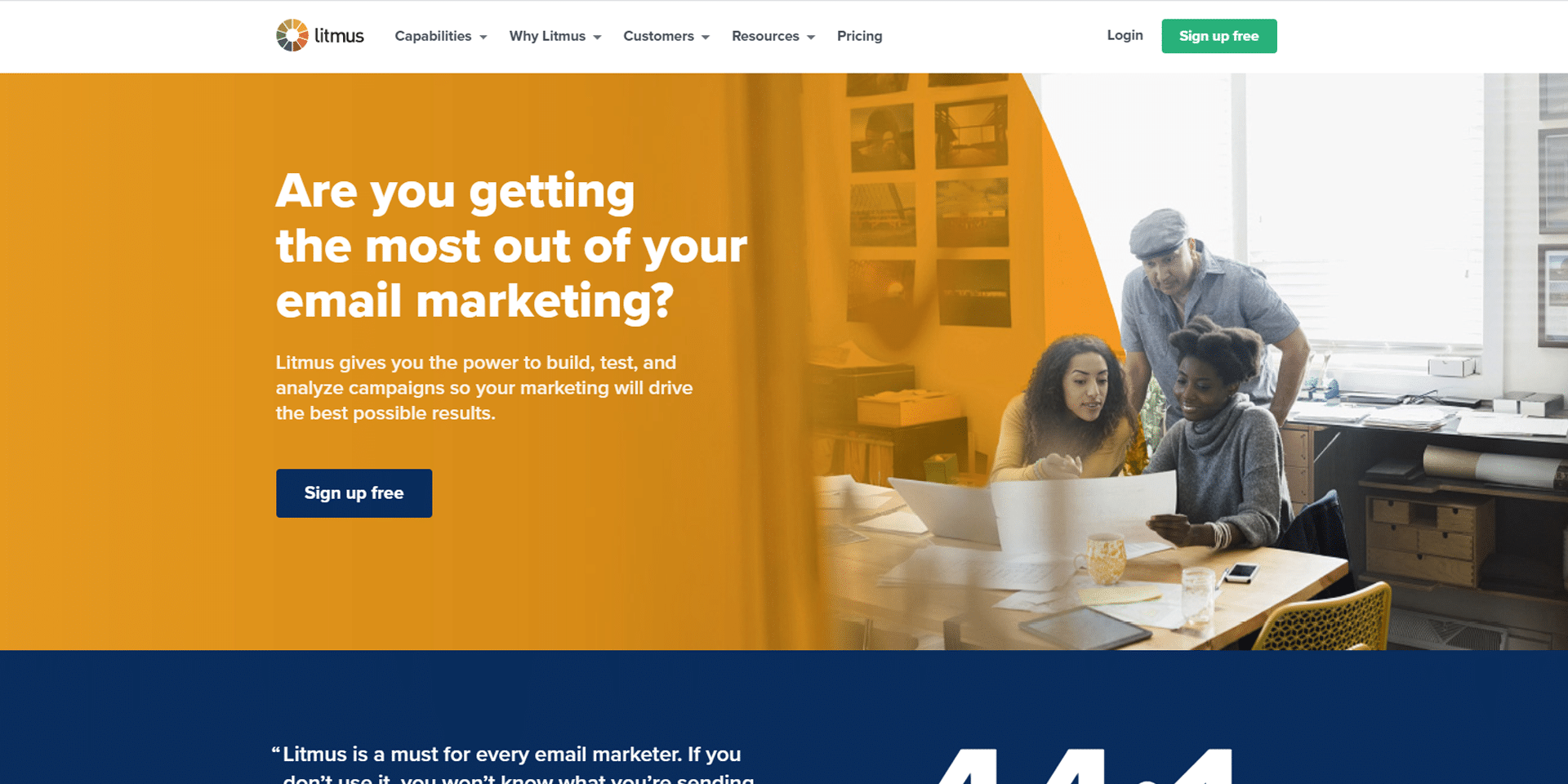The homepage of the website features a clean and organized layout starting with a thin gray line across the top followed by a one-inch white border. Approximately two inches in from the top, there is a circular logo that consists of a white center surrounded by ten colored segments arranged in a clockwise manner. These segments are in shades of brown, red, blue, and burgundy. To the right of this circle, the word "Litmus" is displayed in black text.

Just beneath this are navigation options that include a clickable black space that drops down to reveal links for "Capabilities," "Why Litmus," "Customers," "Resources," and "Pricing." To the right of the navigation links, "Login" is displayed in black text, and next to it, there is a green tab with "Sign Up Free" written in white.

Below the navigation section, a large image spans the width of the page, featuring a warm orange hue overlay. Positioned about two inches from the left, bold white text asks "Are You Getting?" followed by "the most out of your" on the next line, and "Email marketing?" on the subsequent line. Below this headline, there are three lines of smaller white text explaining more details. Further down, a blue tab with "Sign Up Free" written in white stands out.

The background of the image depicts a wall that is visible halfway across the page, adorned with paintings, and a window complete with blinds on the right-hand side. Seated at a table are two African American women who appear to be examining a piece of paper. Standing above them, near the window, is a man dressed in a blue hat and blue shirt. A brown desk is positioned in front of the group.

The bottom two inches of the page feature a dark blue border. Just above this border, in small lettering to the left, it reads "Litmus is a must for everyday email marketer." Adjacent to this, partially cut off by the bottom edge, there is an incomplete segment of text that seems to start with the word "fours."